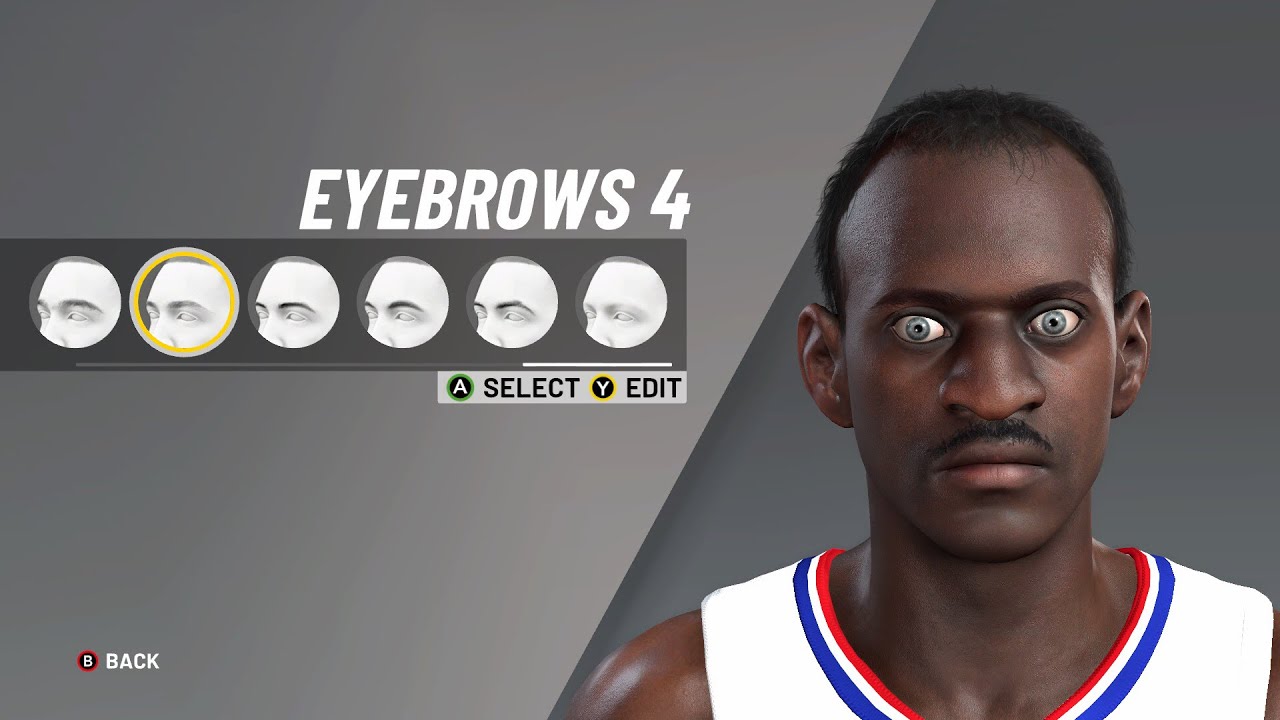The image is a screen capture from a character customization menu within a video game. The screen is split diagonally, creating two distinct sections: the top right in dark gray, and the bottom left in steel gray. The right side features a young male character with unusual gray eyes and a mustache, clad in a sleeveless white basketball jersey accented with blue and orange lines around the neck. His short black curly hair frames his face.

On the left side, white text reads "Eyebrows 4," above a dark gray rectangular banner showcasing six different eyebrow shape options displayed on a Phantom of the Opera-style mask. The second eyebrow option from the left is highlighted with a light yellow outline. Below this banner, a green button with a white "A" is labeled "Select," and a gray button with a white "Y" is labeled "Edit." In the bottom left corner of the screen, a black circle with a red outline features a white "B," accompanied by the text "Back" in white to its right.